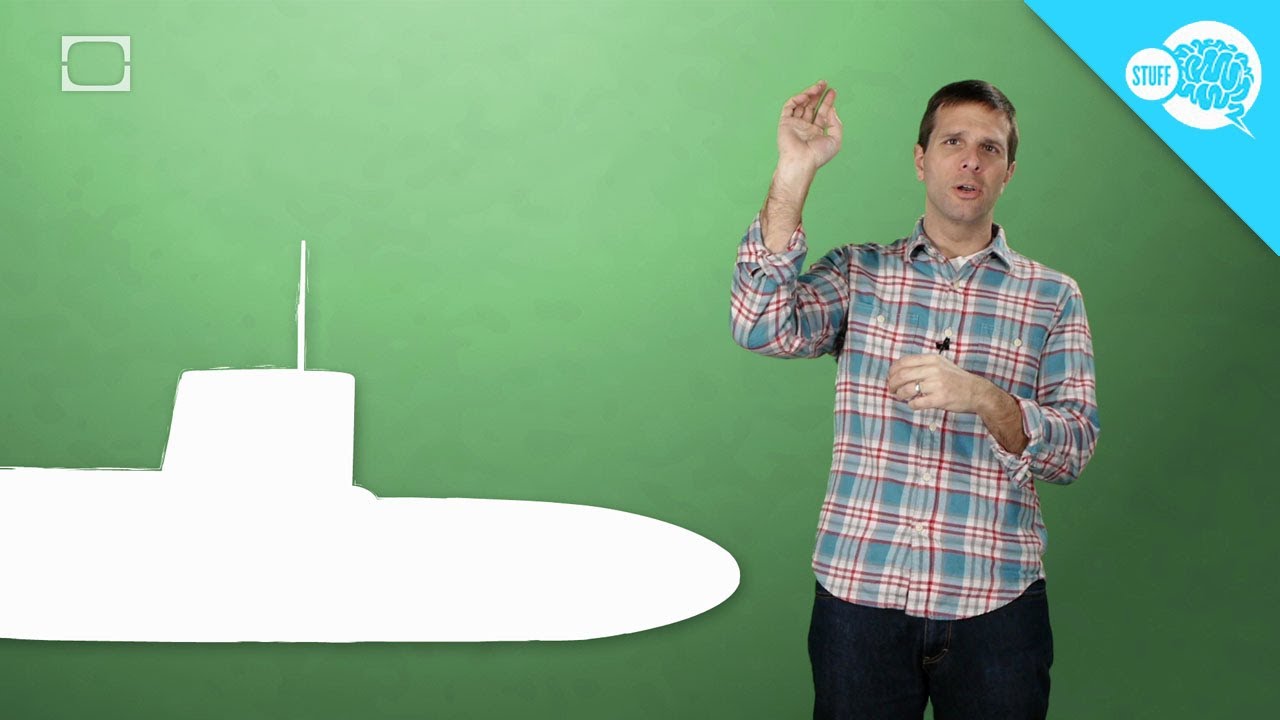The image features a vibrant green background with a distinct triangular blue spot located in the upper right corner. The blue spot is reminiscent of a brain, framed in white, and contains a small white circle inscribed with blue text. On the green portion of the image stands a gentleman who appears to be explaining a detailed illustration. Central to the visual is a meticulously depicted white submarine, complete with an antenna on top. The gentleman, positioned to the side of the submarine, is dressed in a red, white, and blue checkered shirt paired with dark pants. He is captured mid-gesture, with one arm raised and the other resting across his body, as if actively engaging in a teaching moment about the submarine.